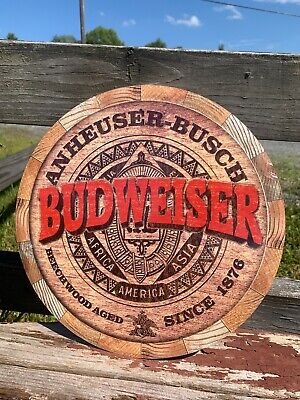The image showcases an outdoor scene with a prominently featured wooden circular sign for Anheuser-Busch Budweiser. The sign, composed of multiple pieces of wood, has the word "Budweiser" boldly written across the center in vivid red letters, while "Anheuser-Busch" and other text, including "Africa, Asia, America" and "Beechwood Aged Since 1876," are engraved in black, mimicking a burnt effect. Below the Budweiser logo is an emblem with ornate designs. This weathered sign leans against a distressed, unpainted wooden fence, which appears grayish and worn. In the background, a sunny day with clear blue skies, a smattering of green trees, an electrical pole with wires, and patches of grass can be observed. There is also a hint of a bench or table, characterized by layers of wood and fading brown paint, situated in front of the fence.